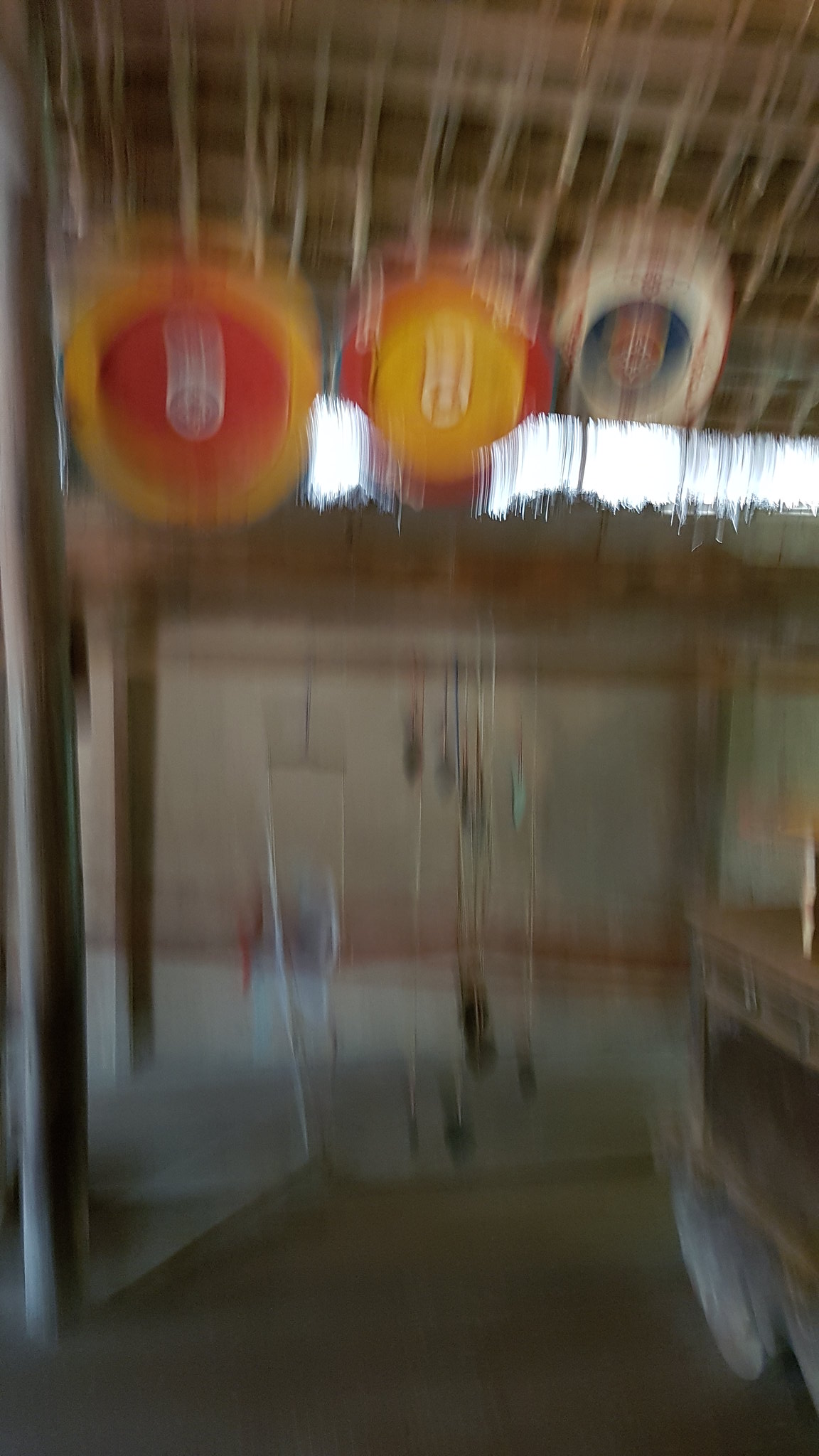This tall rectangular image, despite its blurriness, depicts the interior of a spacious, possibly recreational building or warehouse. The structure is characterized by a high ceiling supported by medium brown wooden beams and cross beams. There are windows in the background, allowing light to filter into the space. Dominating the upper section of the image are three distinct circular objects, reminiscent of targets or shields. The first circle on the left features an orange-yellow outer rim with a red center. The middle circle has an inverse color scheme, with a red outer rim and an orange-yellow center. The third circle is more complex, displaying a combination of white, blue, and red, possibly containing a picture or symbol in its center. These circles are suspended near the ceiling, adding an element of curiosity to the scene. Below these objects, strings or lines hang down. Additionally, there is a box-like object on the right side of the image, potentially on wheels, adding to the enigmatic character of the photograph.